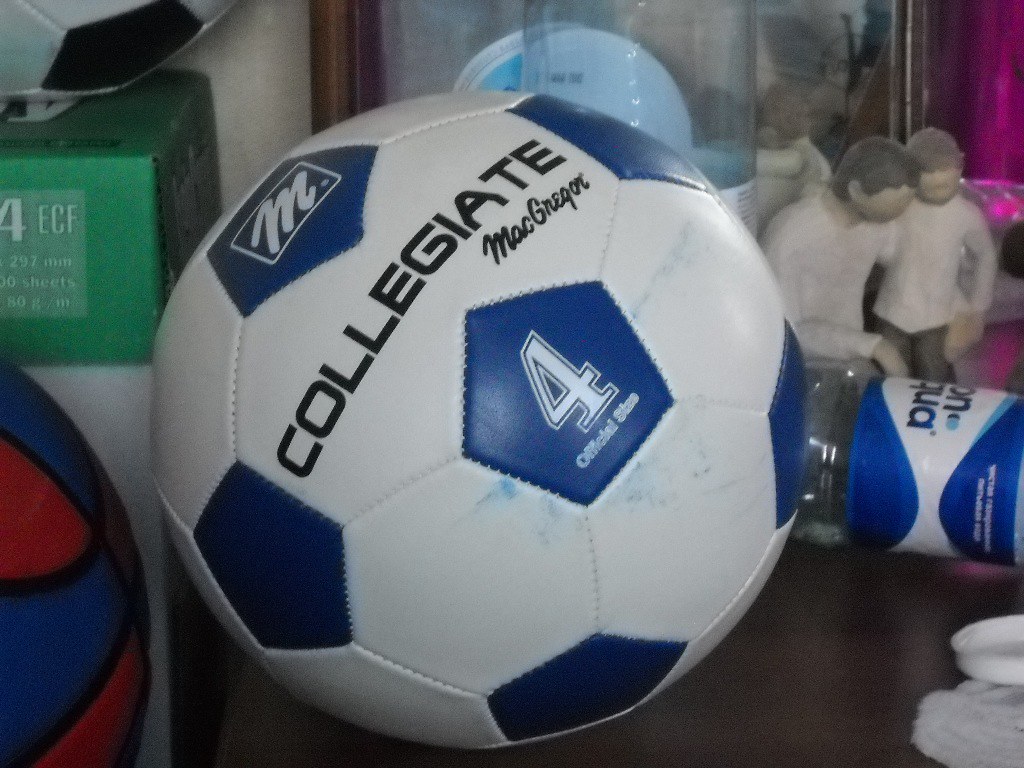The image is a close-up, color photograph of a white soccer ball with royal blue patches in various locations. The ball has black writing across the top that reads "Collegiate McGregor," with a blue hexagon featuring a stylized letter "M" above it, likely the company's logo. In the middle of one of the blue octagonal patches, the number "4" is prominently displayed in white. The soccer ball is situated on what appears to be a table or counter, which is brown and has some decorations. In the background, there are various items, including a water bottle turned on its side with a blue and white label, whose text is unclear. Additionally, two small figurines depicting a man and a boy, both with short hair and wearing white shirts, appear to be hugging. To the side, there is a box containing a red and blue basketball that has not been removed from its packaging.